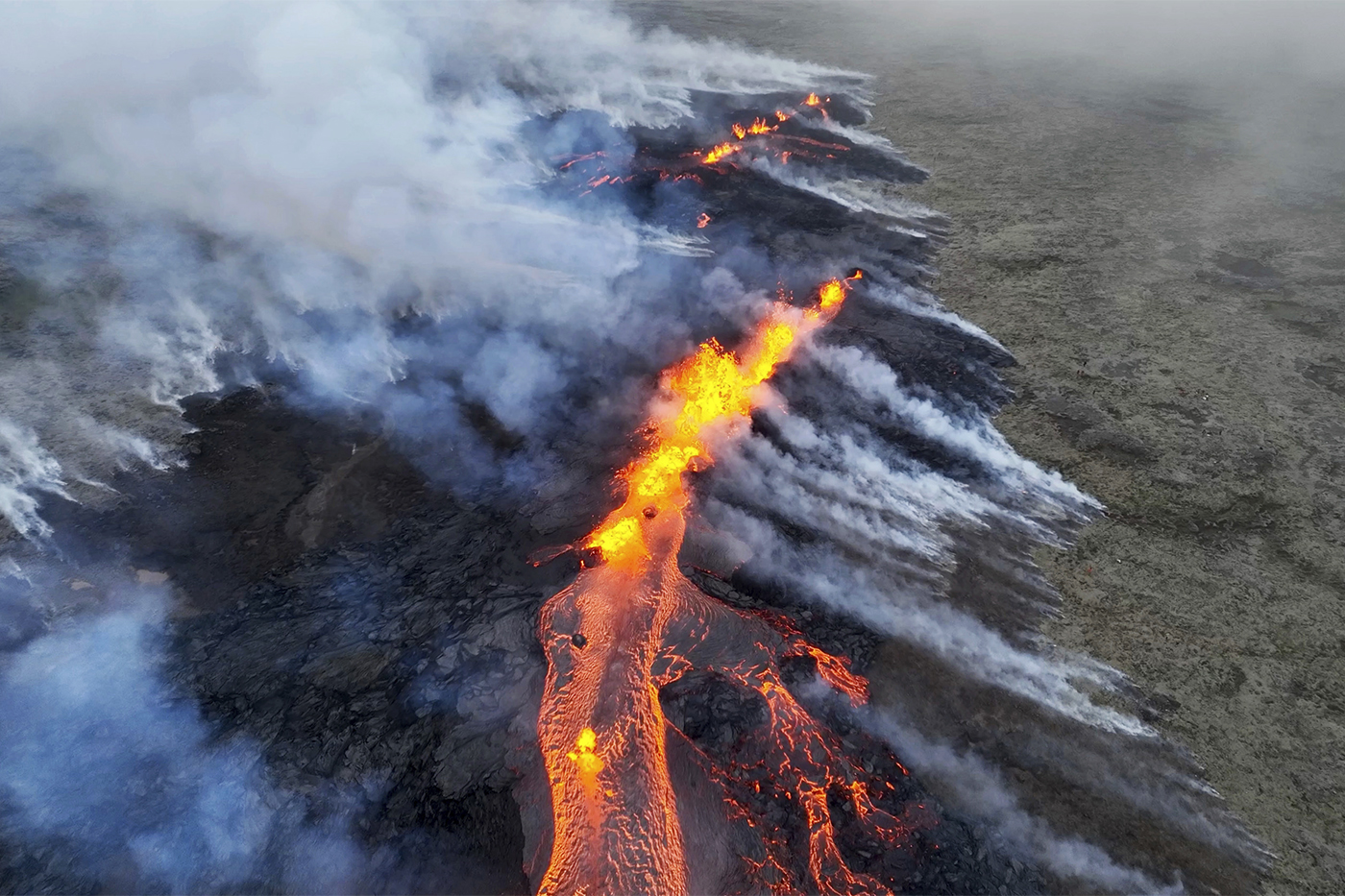This aerial photograph captures the dramatic scene of an active volcanic eruption. The image is split into distinct landscapes: on the right side, a greenish-gray shrub terrain contrasts sharply with the stark, black rocky landscape on the left. Dominating the center of the frame, a vivid, bright orange river of lava flows from the bottom center, curving slightly to the right. Along this molten path are explosive bursts of bright yellow lava ringed by orange and red hues, indicating intense heat. Near the bottom, the lava river is dotted with dark splotches and several tendrils of nearly cooled, black lava outlined faintly in orange. In the top left corner, dense fumes of gray smoke rise upward and drift leftward, a sign of burning vegetation and ash release. Additionally, in the distance towards the top of the frame, another fiery hotspot is visible, smoldering with blackened lava and sporadic bright flames mirroring the lower lava flow. The entire scene, captured in daylight, showcases the contrast between the cooling, cracked, blackened lava and the relentless advance of the vibrant, scorching magma.